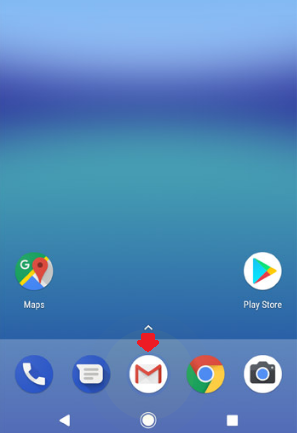Here is a more refined and detailed caption for the image:

---

A screenshot captured from a mobile phone appears to be displayed upside down. The screen transitions from a light blue at the top to a darker blue at the bottom, creating an ombre effect. 

At the upper edge (which is actually the bottom due to the upside-down orientation), a series of icons are visible. On the left side, there is a Google Maps icon. To the far right, there is a Play Store icon in Google's characteristic colors. 

Beneath these icons, a horizontally aligned bar in lighter blue spans the width of the screen. In the center of this bar, there's a red downward-pointing arrow. 

To the left of the arrow, a circle icon with an "M" inside, possibly representing 'Mail', is seen. Left of this, there is another circle icon displaying a piece of notepaper on a blue background. Adjacent to it is an icon featuring a white phone on a blue circle.

On the right side of the red arrow, a circle with Google's colors is present, and further right, another circle with a camera icon can be seen.

At the absolute bottom (or top, if correctly oriented), typical navigation icons of a smartphone are displayed: a small triangle, a circled dot, and a small square.

Despite the upside-down display, the apps' icons are oriented correctly, adding to the confusion.